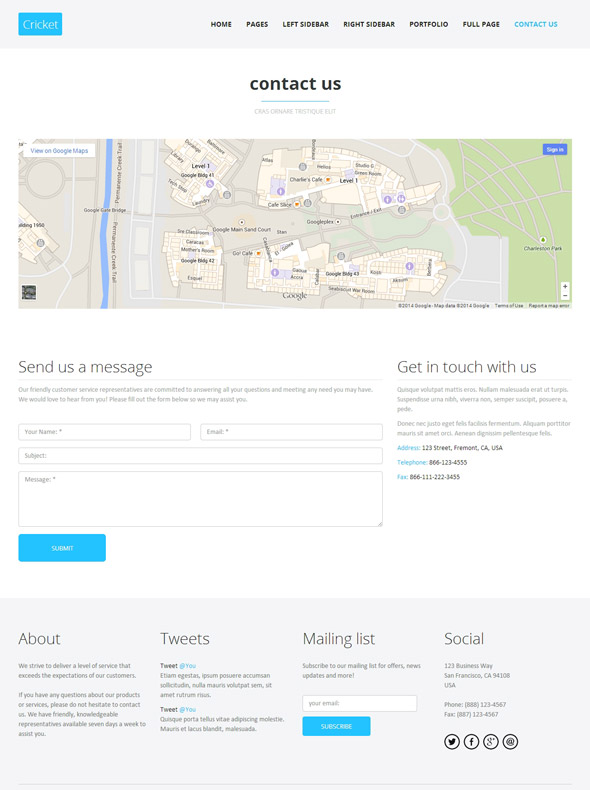The image depicts a well-organized website interface with a blue button labeled "Cricket" located at the top left corner. To the right of this button are several black headings, which include "Home," "Pages," "Left Sidebar," "Right Sidebar," "Portfolio," "Full Page," and a smaller blue link labeled "Contact Us." The blue color of "Contact Us" indicates that this is the current page being displayed. 

Prominently centered below the heading is the text "Contact Us" in a much larger font. Directly beneath this title is an interactive map with zoom in and out options on the right-hand side. Below the map, on the left side, is a "Send Us a Message" box where visitors can input their name, email address, and a short message; a blue "Submit" button allows them to send this information to the website administrators. 

On the right side of the contact section, alternative contact methods are provided, including the physical address, telephone number, and even a fax number. Below these contact details, the page features a large grey panel divided into general headings such as "About," which provides details about the site, "Tweets," "Mailing List," and "Social." Directly below the "Mailing List" heading is a small blue button, likely for subscribing to updates. The website is designed with a clear and user-friendly layout, making navigation intuitive and straightforward.